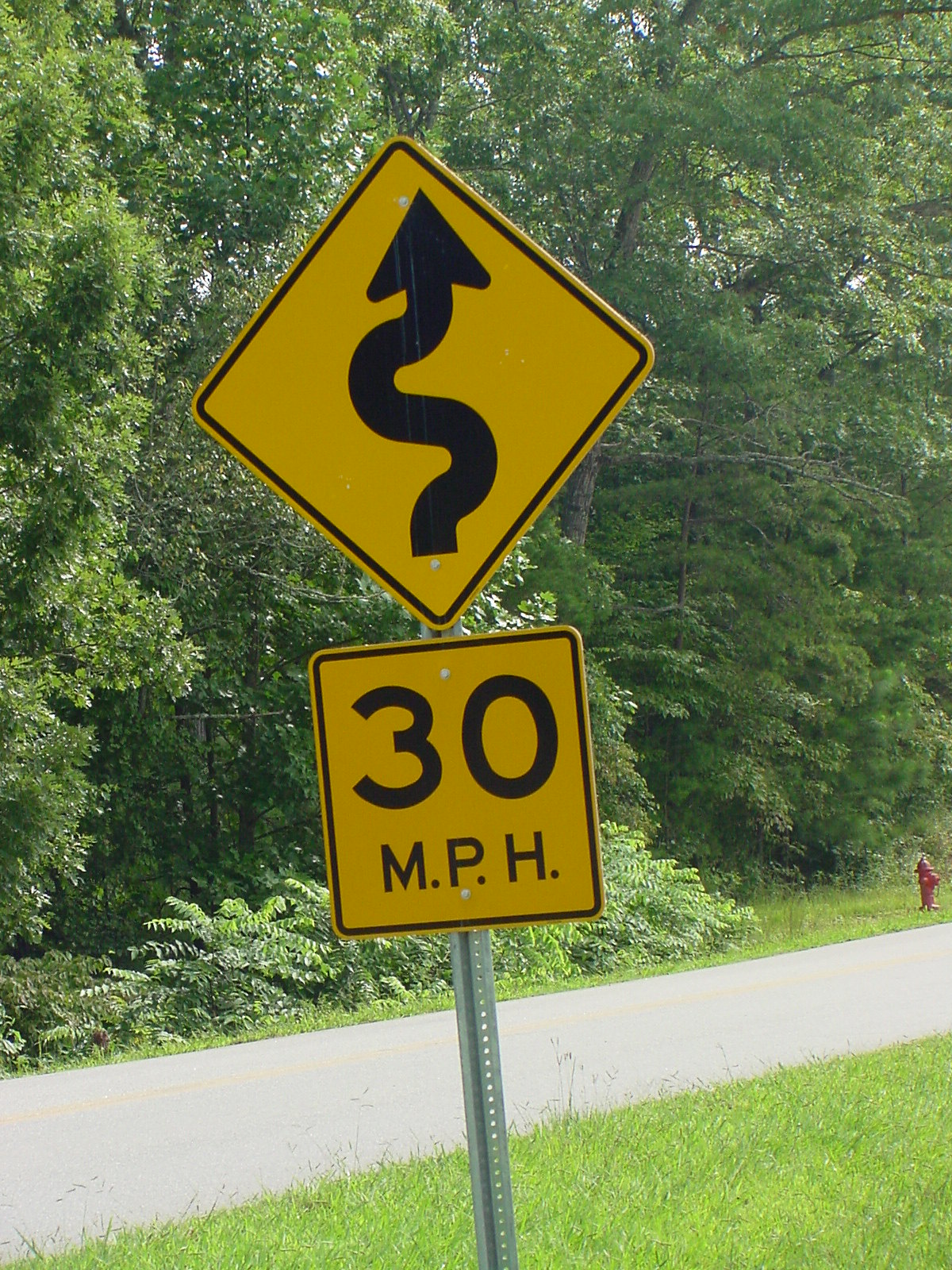The image captures a street scene dominated by a prominently featured street sign positioned in the center. The sign is mounted on a corrugated metal pole with numerous holes. The top section of the sign is a yellow square turned on its point to resemble a diamond shape, outlined in black, and it displays a black, squiggly arrow indicating a winding road ahead. Directly below this is another yellow square sign, this one set flat, which reads "30 MPH" in bold black letters.

The background of the image offers a picturesque view of a road flanked by grassy areas. On the right side, about a third of the way up, there is a red fire hydrant. The far distance reveals a lush panorama of shrubs and tall trees, forming a heavily wooded area that obscures much of the sky. The greenery extends across the image, providing a natural, verdant backdrop to the functional yet prominently placed street sign.